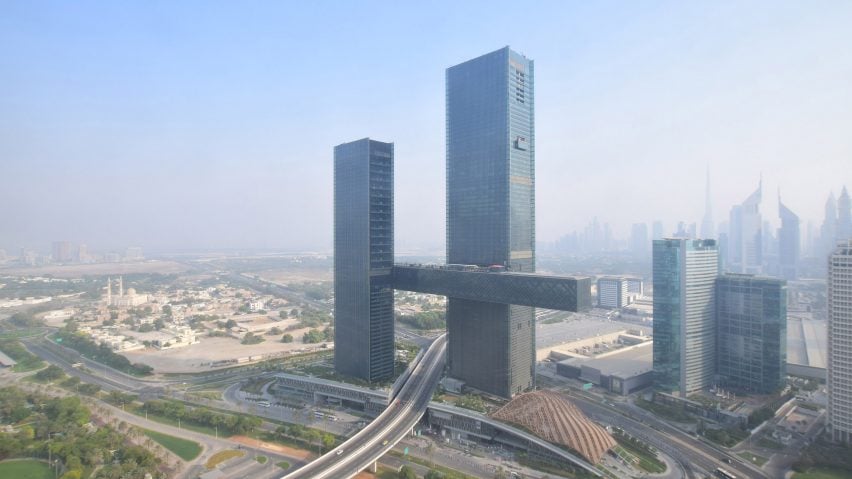This horizontal, aerial photograph captures an expansive view of a bustling cityscape on a hazy, blue-sky day. Dominating the center of the image are two prominent skyscrapers: the one on the left is shorter, while the one on the right is taller and features a distinctive horizontal section that connects to its base, resembling a bridge-like structure. Between these buildings, a freeway runs through the scene, with visible cars traveling along its gray asphalt. To the right of the main skyscrapers, several smaller office buildings and additional skyscrapers extend into the background, forming a sharp, pointy skyline. The top of the sky transitions from blue to a pinkish-white gradient, suggestive of pollution. The photo is framed with lush greenery, including trees and grassy areas, particularly noticeable in the bottom left corner, adding contrast to the urban environment. The overall scene is a typical but intriguing view of a city, albeit slightly obscured by the hazy atmosphere.